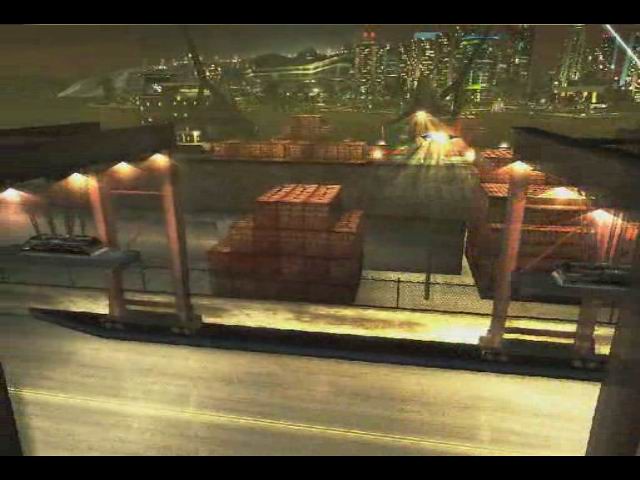The image features graphics reminiscent of a video or computer game. In the foreground, there's a street marked by a pale yellow line. An industrial area dominates the midground, guarded by dark-colored fencing. Beyond the fence, stacks of orangey-brown cargo boxes come into view, mingling with whites that cast a subtle yellow hue. On one side of the image, dark-colored cars are parked, further accentuating the industrial vibe. The background reveals additional cargo and a distant city skyline adorned with skyscrapers. These high-rise buildings are bathed in a soft amber and white light, creating a grainy, slightly distorted ambiance.